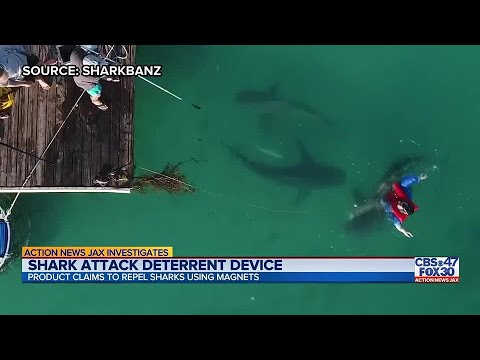The image is a screenshot from a television broadcast on the news station CBS 47 FOX 30. The broadcast features a segment titled "Action News Jax Investigates," with the specific investigative report labeled "Shark Attack Deterrent Device: Product Claims to Repel Sharks Using Magnets." The image shows a person in deep, murky green waters, wearing a blue shirt and a red life jacket. Several dark silhouettes of sharks can be seen swimming beneath the surface near the person. In the background, a brown wooden pier extends over the water, with people standing on it. These individuals are holding fishing poles, possibly testing the magnetic shark deterrent device. At the very top of the screen, the source is cited as "shark bands." The scene captures an experimental setup intended to demonstrate the effectiveness of the shark repellent device.